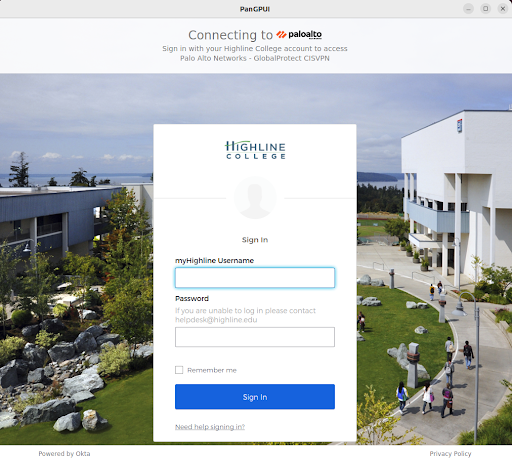Captured from the Highline College website, this image prominently features the college campus as seen from an elevated vantage point, perhaps atop one of the buildings. In the foreground, students stroll along the campus sidewalks, enveloped by a lush array of trees. The skyline in the distance is overcast, with clouds casting a muted light over the scenery. The campus itself boasts modern architecture, with some buildings featuring large windows, while others stand out due to their intricate and beautiful design.

The screenshot also includes an online interface, likely for accessing a secure network. At the very top, a message reads "Pan G-P-U-N-I, Connecting to Palo Alto," followed by instructions to "Sign in with your Highline College account to access Palo Alto Networks GlobalProtect." Below this header, the interface displays a form for Highline students, inviting them to sign in with their Highline College username and password. The input fields are bordered by a distinctive teal color. Additional texts prompt users: "If you are unable to log in, please contact the Help Desk." Alongside this, there are checkboxes for "Remember Me" and a blue button labeled "Sign in."